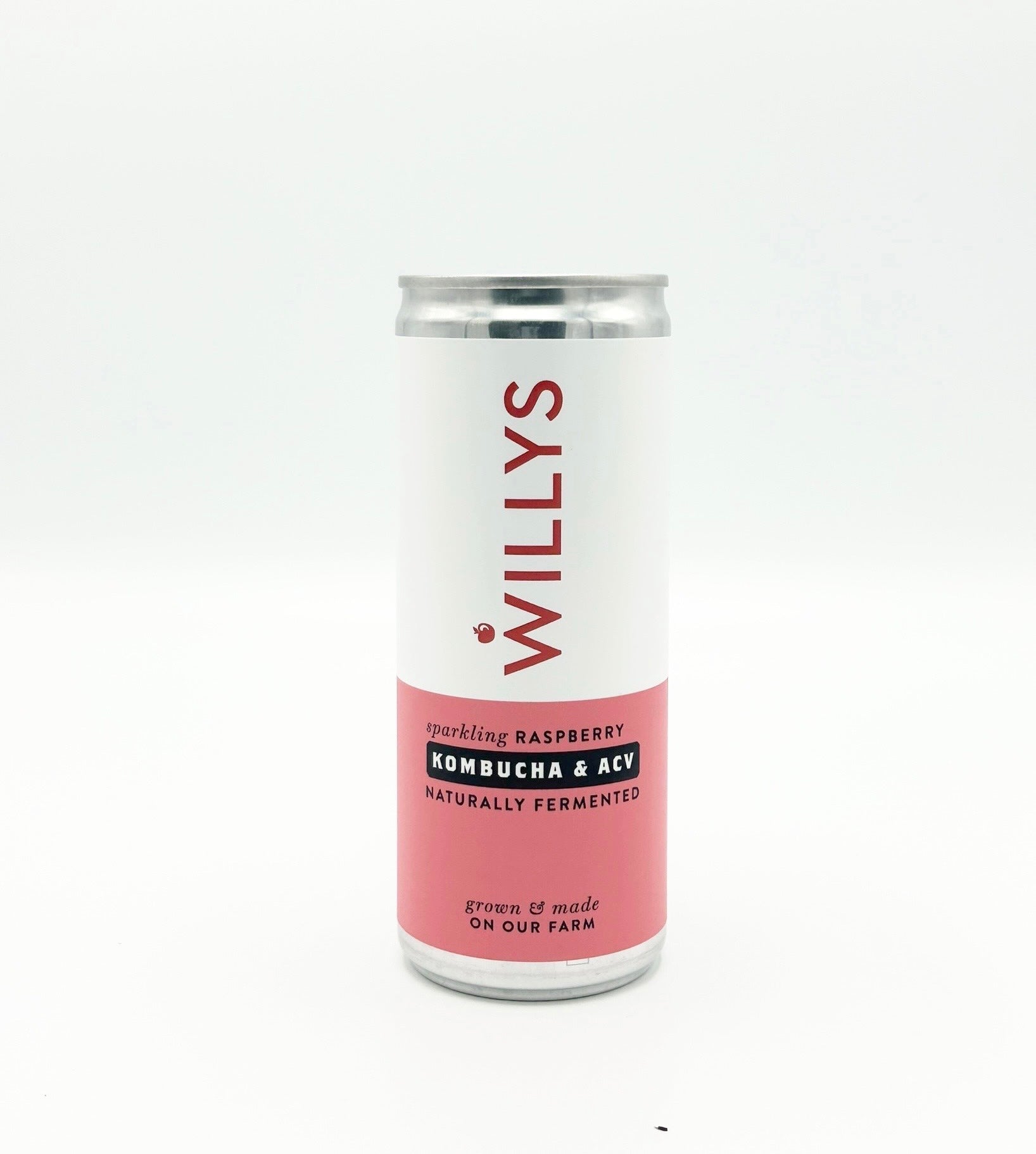The image depicts a tall, slender aluminum can of kombucha set against a plain white background. The can is stylishly designed, resembling those typically used for alcoholic beverages like White Claw. The top half of the can's label is white with the brand name "Willys" written in bold, red horizontal lettering, featuring an apple graphic above the "W." The lower half of the label transitions to a blush pink shade and contains several descriptive texts: in black lettering, it reads "sparkling raspberry kombucha and ACV," followed by a smaller text stating "naturally fermented." At the very bottom, also in black text, it says "grown and made on our farm." The can's sleek silver base contrasts with the vibrant label, making the branding and product details stand out.